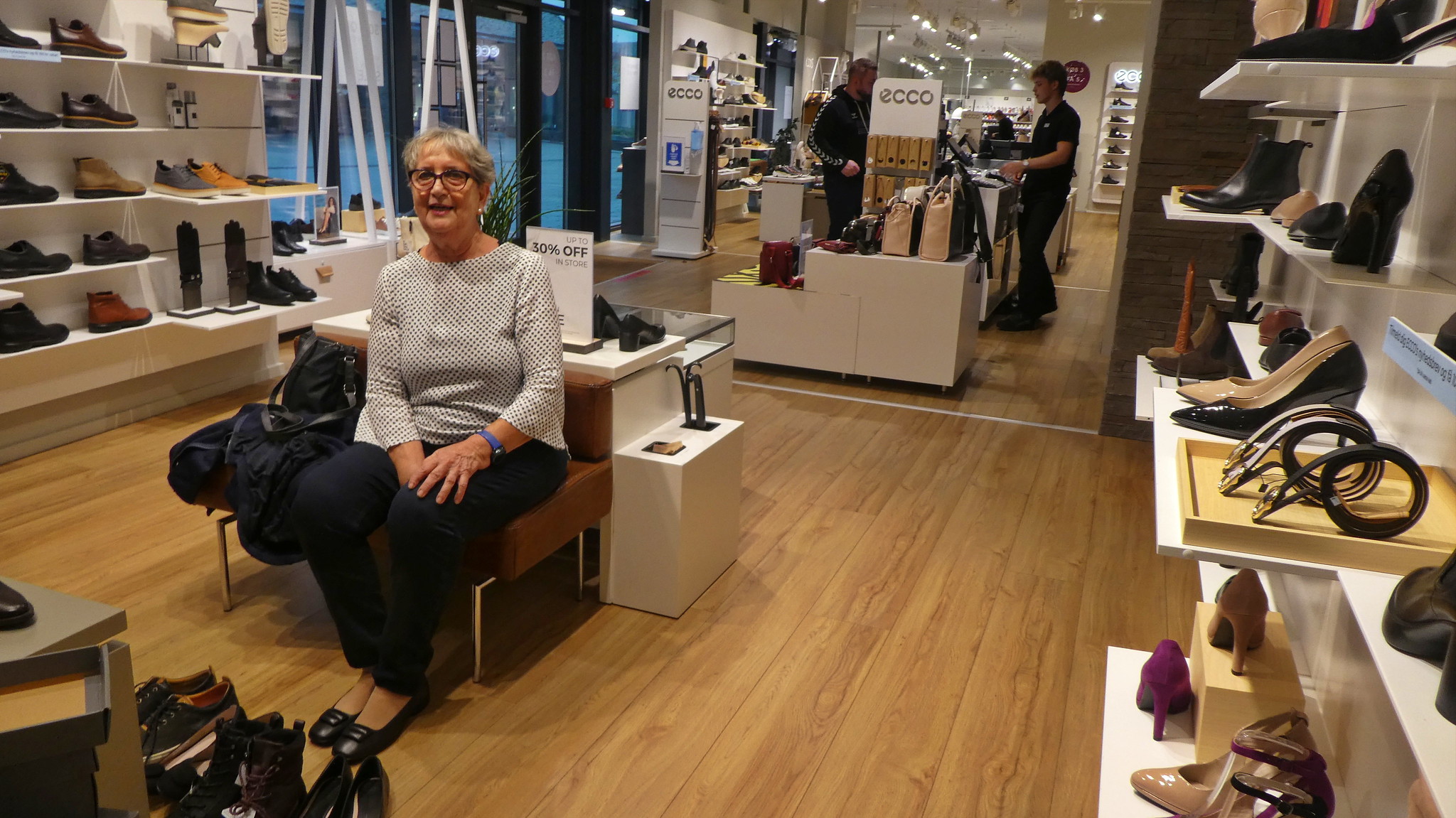In the image, a woman with gray hair and black-framed glasses is seated slightly off-center to the left on a brown bench in a shoe store with hardwood flooring. She is wearing a white shirt with black pants and black shoes, and has a light blue wristwatch on her left arm. In front of her and to her left are various shoes in an array of colors, including orange, black, tan, blue, and magenta, displayed on shelves and the floor. A bag is next to her on the bench. Behind her, there is an open door and window, which provide some natural light. To the top right of the image, a man dressed in a black t-shirt and black pants is at a cash register, assisting another man on the other side of the counter. The store also features signs that read "ECCO" and "30% off," and has a mix of light brown, black, gray, and other colorful elements contributing to the lively atmosphere.